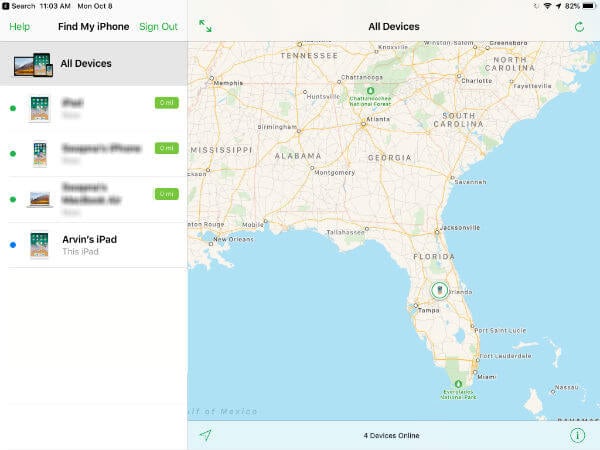This image is a detailed screenshot from a device locator application, captured at 11:03 a.m. on Monday, October 8th. At the top, the interface features a black 'Search' bar, along with the time, date, Wi-Fi signal, and battery level at 82%. On the left, green text options for 'Help' and 'Sign Out' are present, while 'Find My Phone' is highlighted in larger, darker black print. Below these options, there are sections labeled 'My Devices' and 'All Devices,' listing four items. The first three device names are obscured, showing only their icons—an iPhone, an iPad, and a laptop. The fourth device, 'Arvind's iPad,' is clearly visible, marked as 'This iPad' and currently selected.

The right side of the screenshot displays a map covering several states including Tennessee, North Carolina, South Carolina, Georgia, Alabama, Mississippi, and Florida, with major cities prominently labeled. Further down the interface, a green text label indicates a park, and at the bottom of the screen, there is a note stating '4 devices online,' accompanied by a green circle containing the letter 'I.'